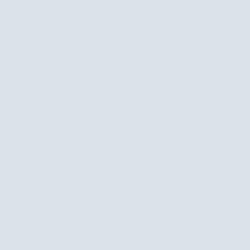The image appears to be a blue-gray square with no discernible features, text, or images. The square occupies the entire frame, making it difficult to estimate its resolution. This could potentially be a result of an image load failure from the server or simply an improperly taken screenshot. There are no additional elements within the image to provide further context or details.